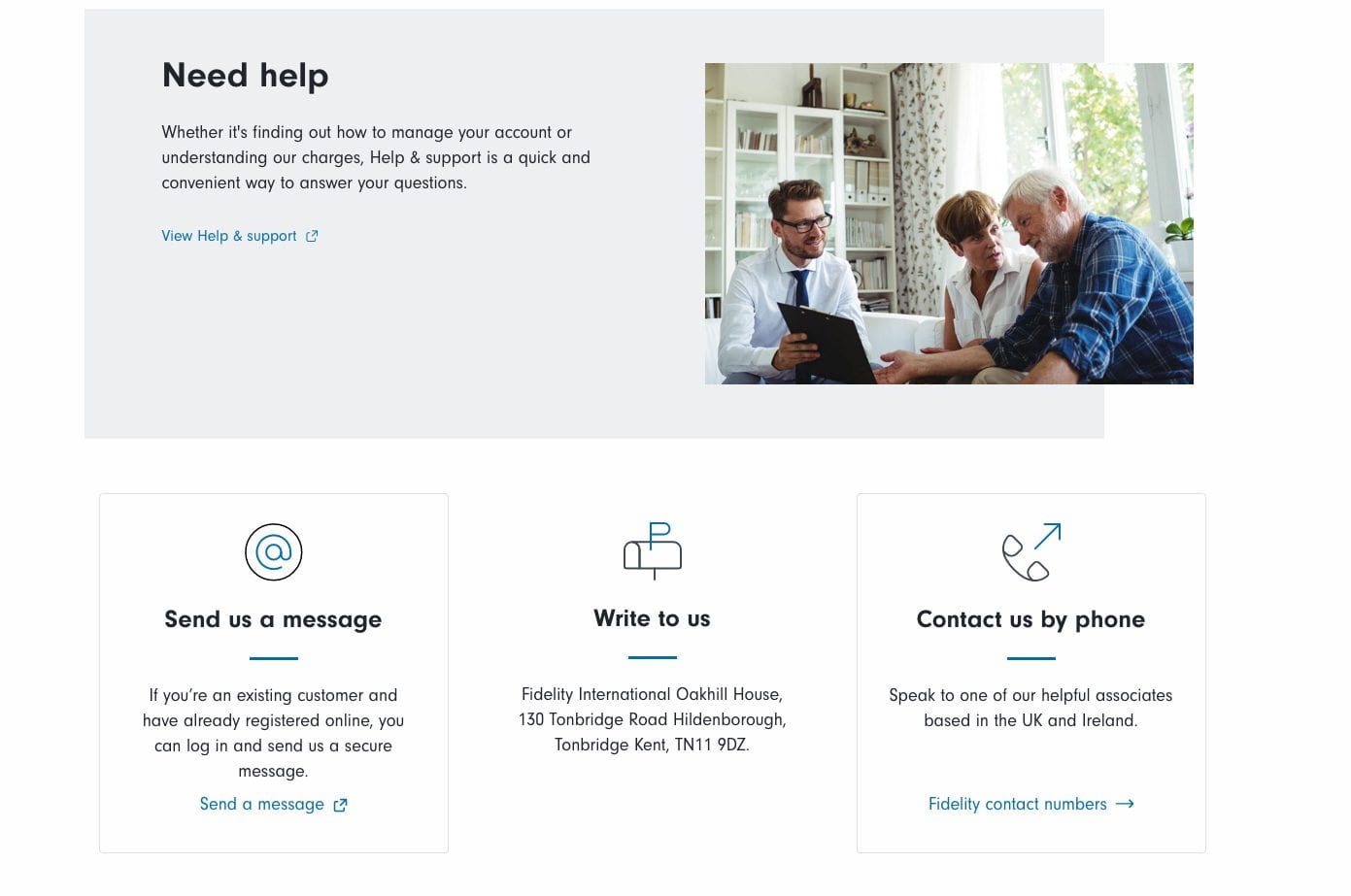The on-screen image features a light gray box with helpful information for users. 

- On the left-hand side, the text reads: "Need help? Whether it's finding out how to manage your account or understanding our charges, help and support is a quick and convenient way to answer your questions." Beneath this text, there is a clickable blue link labeled "View Help and Support," which directs users to the help and support page.

- On the right-hand side of the image, there is another square box featuring a photograph of a Caucasian man holding a laptop, demonstrating something to a Caucasian couple. The woman has short brownish hair, and the man has gray hair. The trio appears to be intently looking at the screen of the laptop while seated on a couch.

- Below the photograph, two smaller boxes offer further contact options. The first box states: "Send us a message. If you are an existing customer and have already registered online, you can log in and send us a secure message." This text is accompanied by a clickable blue link that says "Send a message," which directs users to the messaging portal.

- The next box reads: "Write to us," followed by the company's physical mailing address. Additionally, it provides information on how to contact the company by phone.

Each section is designed to guide users towards the appropriate channels for seeking assistance or making contact.